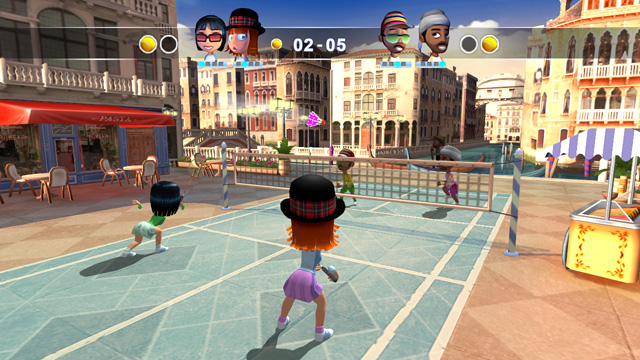Screenshot from what appears to be a Wii game, featuring an exhilarating tennis match set in a charming, cartoonish environment. The match showcases mixed doubles, with two girls and two guys on each team. The men’s team is currently leading, as indicated by the score of 5-2. The vibrant setting resembles a picturesque European locale, reminiscent of Italy or Paris, complete with quaint two- or three-story buildings that seem to serve as both businesses and residences. Adding to the lively atmosphere, a hot dog stand is visible nearby. The characters are dressed in unique and colorful costumes, enhancing the whimsical and engaging feel of the game.